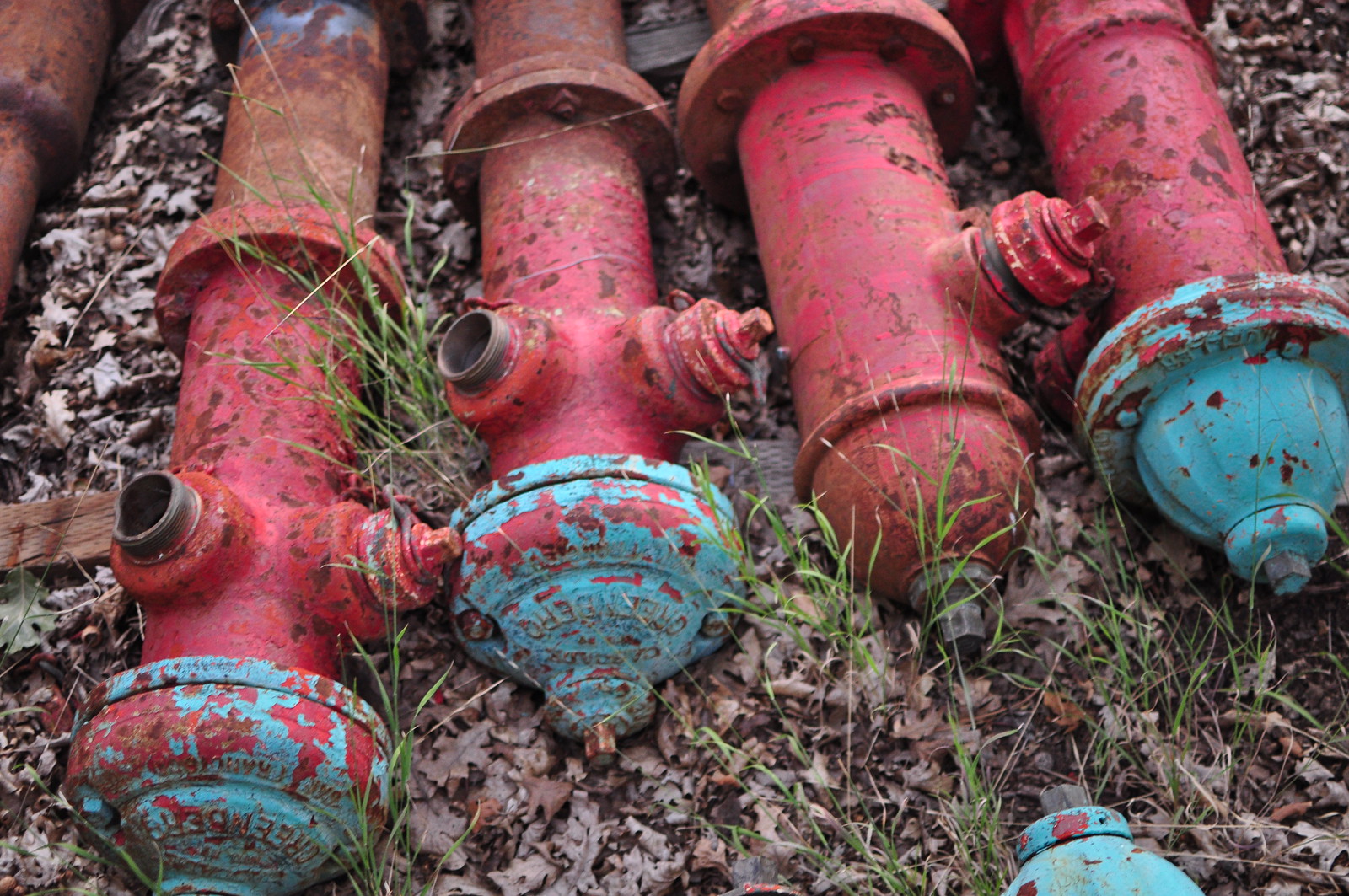This detailed image showcases five old, red fire hydrants with blue caps, no longer in service and lying on a bed of brown leaves with some patches of green grass. These hydrants, irregular with two to three hose fittings on the sides, are arranged next to each other on the ground. Each hydrant is mounted to rusty iron pipes that once anchored them into the ground. The blue paint on the caps appears faded and peeling, exposing the red beneath. The second hydrant from the right is missing its cap, but a blue cap is visible lying off to the side. The hydrants exhibit signs of age and wear, emphasizing their removal and disuse.